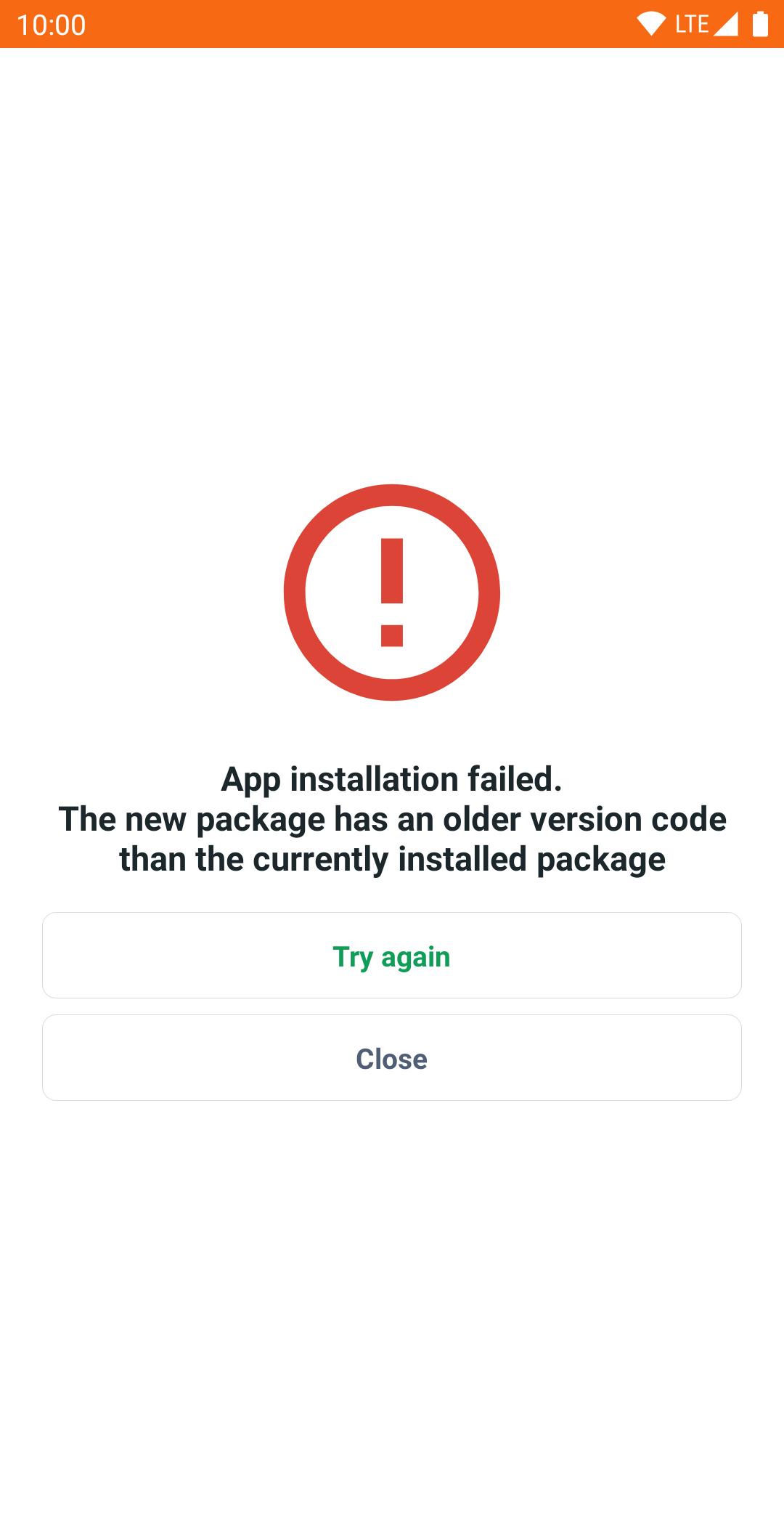The image on the smartphone screen features an orange banner at the top, where the clock displays "10:00" on the left side. On the right side of the banner, it shows indicators for a strong LTE network connection, full Wi-Fi signal strength, and a fully charged battery.

Below the banner, there is a large white panel occupying most of the screen. Centrally positioned within this panel is a red circle with a red exclamation mark inside, signifying a warning. Directly under this warning symbol, in black text, is a message stating: "App installation failed. The new package has an older version code than the currently installed package." 

Beneath the message, there are two white buttons for the user to choose from. The first button, on the left, has green text that says "Try Again." The second button, on the right, has grey text that says "Close." The screen is otherwise devoid of any additional elements, focusing entirely on the warning message and the two interaction options.